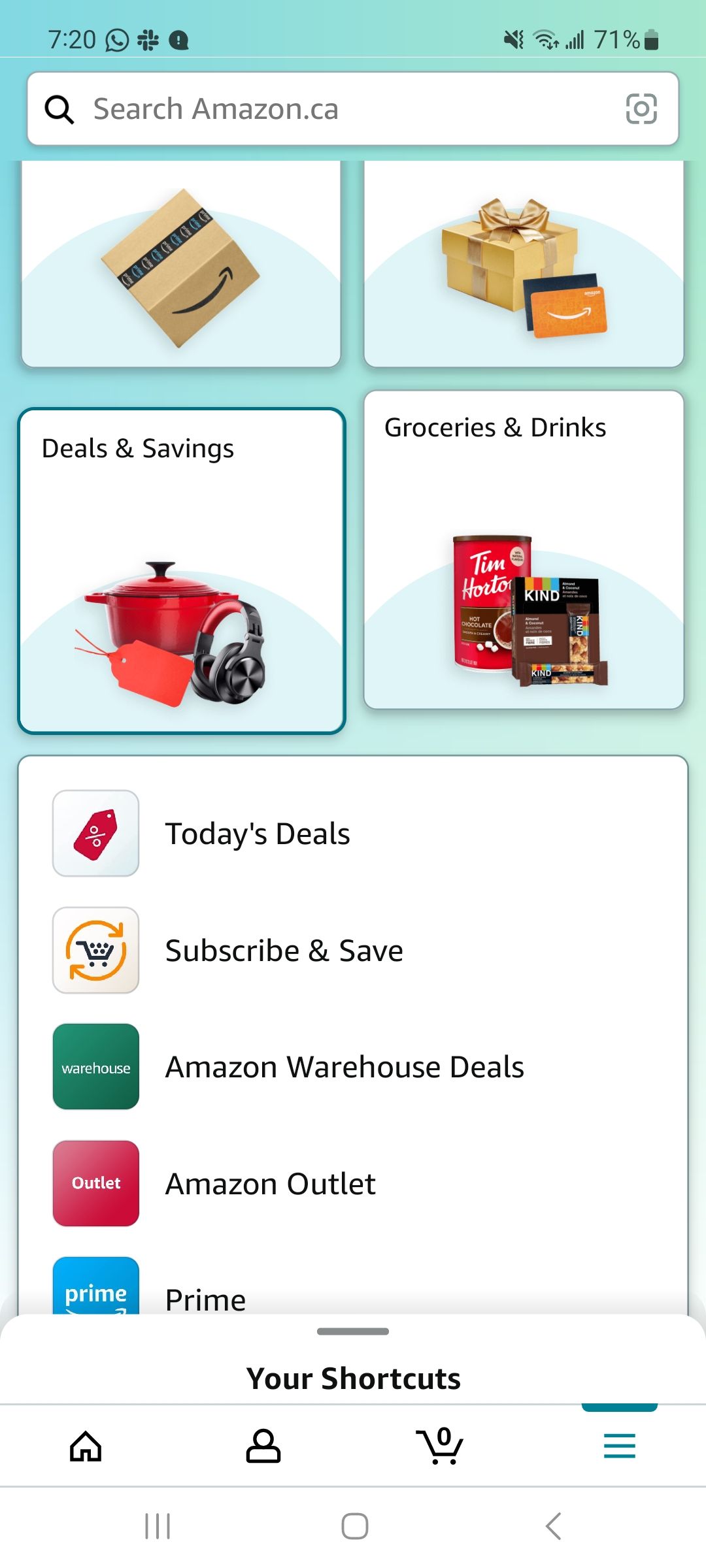The image depicts a screenshot of the Amazon app on a smartphone. The smartphone display shows a green background. Let's break down the details:

- **Top Left Corner:**
  - The time is displayed as 7:20.
  - The WhatsApp icon is visible.

- **Top Right Corner:**
  - Reception and Wi-Fi signal icons are present.
  - The sound is turned off, as indicated by the silent mode icon.
  - The battery percentage shows 71%.

- **Below the Status Bar:**
  - A white search bar labeled "Search Amazon.ca" is centered at the top.

- **Main Interface:**
  - The screen shows various sections organized into boxes.
  
  - **First Box (Left):**
    - Contains an image of a brown Amazon box.

  - **First Box (Right):**
    - Displays a golden gift and an adjacent orange gift card.
  
  - **Second Box (Left):**
    - Titled "Deals and Savings" and shows images of a red pot, a red sale tag, and headphones.
  
  - **Second Box (Middle, Right):**
    - Section labeled "Groceries and Drink" with an image of a red container.
  
  - **Second Box (Far Right):**
    - Titled "Kind," displaying images of snack bars.
  
- **Below the Boxes:**
  - A white area with various categories listed:
    - "Today's Deals"
    - "Subscribe and Save"
    - "Amazon Warehouse Deals"
    - "Amazon Outlet"
    - "Prime"
    - Each category has an accompanying icon.
  
Below this section, another header titled "Your Shortcuts" is present, with icons representing a house, a person, a cart, and three vertical green lines.

The detailed layout and specific elements provide a comprehensive snapshot of the Amazon app interface as seen on the user's phone.